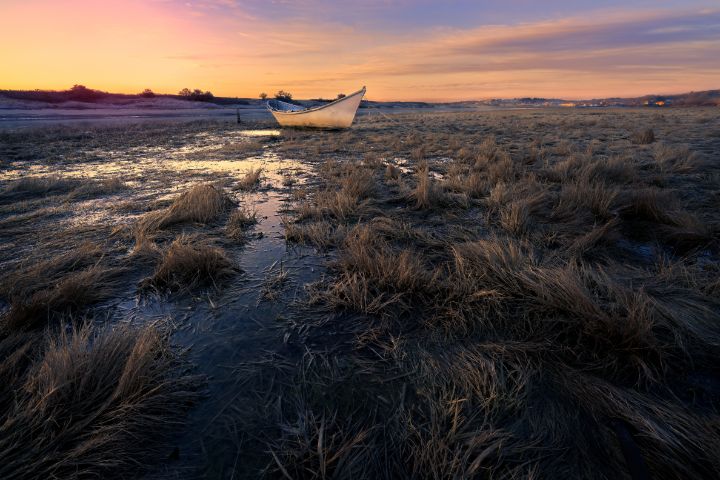This photograph captures a serene, marshy landscape at dusk, with a sky bathed in shades of pink, purple, and blue. The expansive scene primarily consists of a muddy field interspersed with tufts of seagrass and patches of shallow water, creating an almost mosaic-like texture. Towards the back of the composition lies an old-fashioned, white wooden rowboat with a high bow and stern, stranded and resting on the moist ground, indicating a receding tide. In the distance, beyond the boat, the horizon features a beachy area, and subtle city lights possibly glimmer, adding a touch of human presence to the tranquil, natural setting. The overall image has a slightly stylized appearance, enhancing its dreamlike quality.